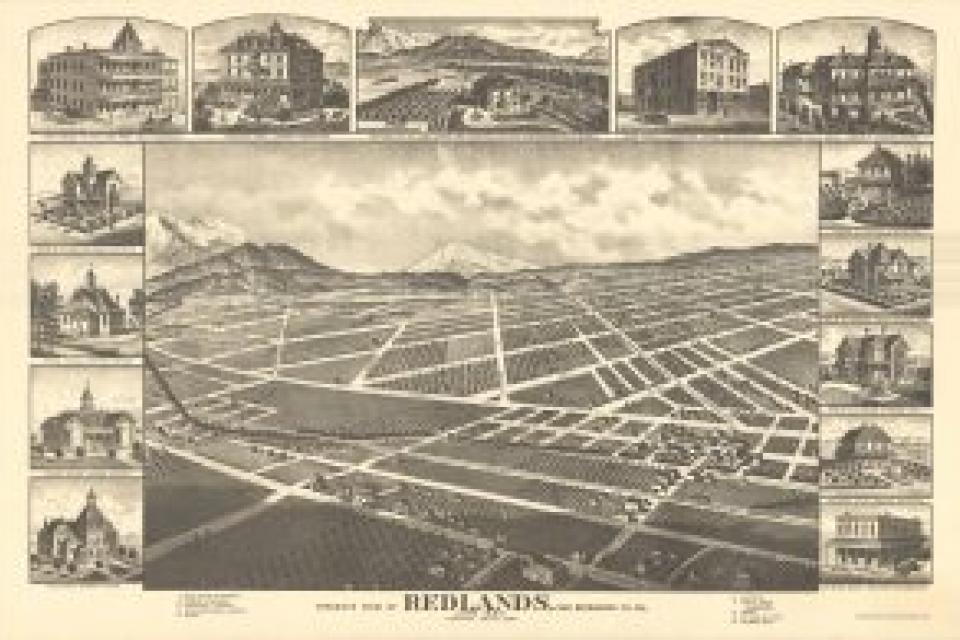This vintage, horizontally aligned poster features a pixelated cream-colored background and depicts a hand-drawn city grid, likely representing an old town named Redlands. The central illustration portrays a semi-rural landscape with a partially cloudy sky and mountainous terrain—two prominent hills to the left, one smaller on the right, and a division of land into numerous parcels by vertical and diagonal lines. The scene includes small houses and other structures along these plotted streets.

Surrounding the main illustration, the poster is bordered by smaller, horizontally aligned rectangles depicting key buildings and locations within the city. These include gabled buildings with triangular roofs and central towers, as well as various single- and multi-story structures like houses, apartments, and possibly a church, all arranged in two columns on either side of the central image.

The poster, rendered in black, white, grey, and soft pink hues, seems to date from the late 1800s to early 1900s. This is suggested by the architectural styles and the flattened, blocky font resembling a squished Times New Roman. At the bottom, the word "Redlands" is legibly centered beneath the landscape, surrounded by faintly readable text blocks on either side and additional fine text below the landscape image. The aged appearance of the paper indicates its historical value.